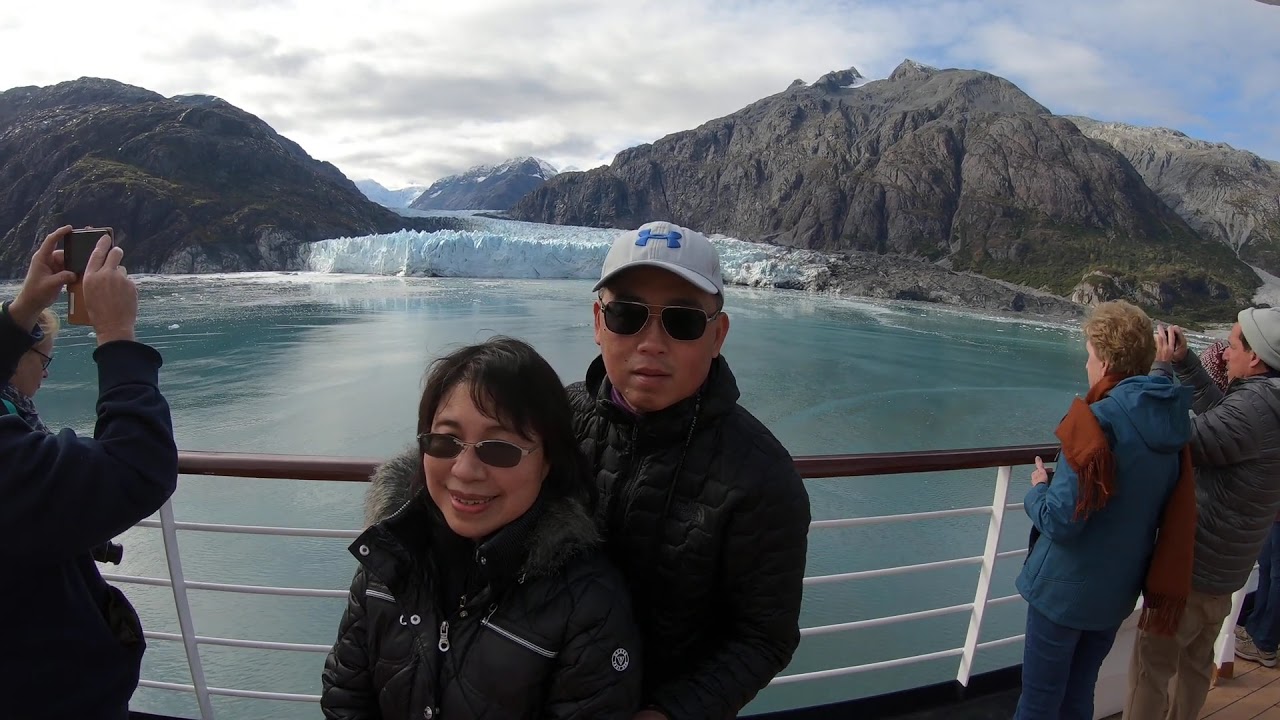In this detailed color photograph, two people are the central focus, standing in front of a wood and white metal railing on a cruise ship deck. The woman on the left wears a puffy black jacket with a fur-lined hood, dark sunglasses, and has dark black hair, while smiling at the camera. The man to her right, posing with his arms around her, has a more serious expression and is wearing dark black glasses, a gray hat with a blue Under Armour logo, and a black jacket. Both are staring directly at the camera, which they appear to be holding as it is a selfie in landscape orientation.

Behind them is an expansive view featuring bright crystal blue water, indicating it is possibly an ocean or bay. Prominently in the water is a large block of ice or glacier, flanked by brown rocky hillsides and further back, snow-covered gray mountains under a bright blue sky with white clouds. To the left and right of the couple, other cruise passengers can be seen taking photographs of the stunning scenery, emphasizing the cold climate. The scene beautifully captures the juxtaposition of vibrant and serene natural elements, framed by the ship's railing and bustling activity of fellow travelers.